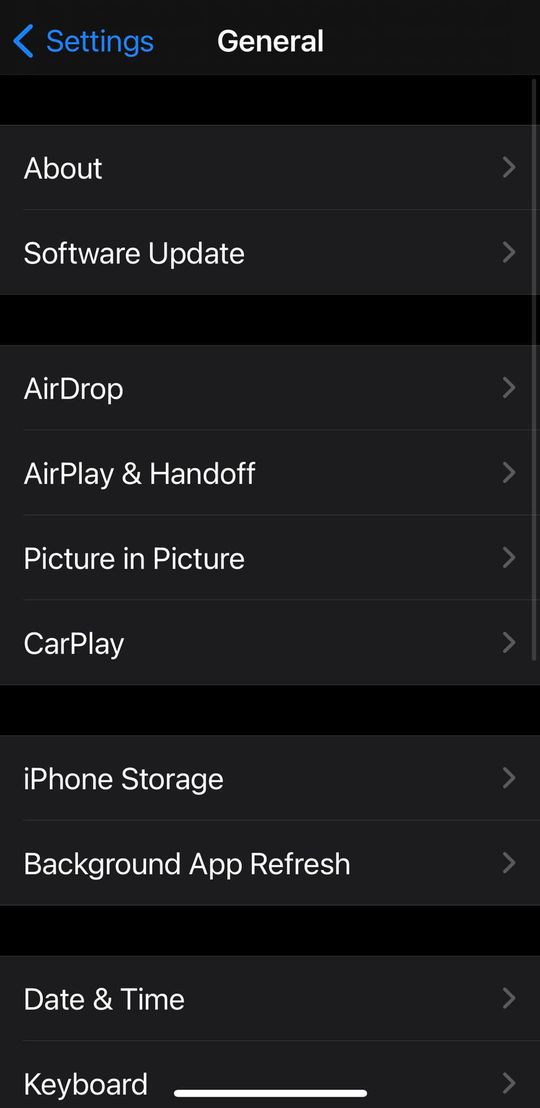This image is a screenshot taken from a cell phone, displaying the "Settings" menu in its "General" section. 

At the top of the screen, the word "Settings" is prominently displayed in blue, next to a left-pointing arrow. Below this, the word "General" appears in white text. The entire screen features white text on a black background, with subtle variations in the black shade creating rectangular highlights around each menu item for better visibility.

The screen lists several options in neatly separated sections:
1. **About** - An arrow pointing to the right accompanies this option.
2. **Software Update** - This item is directly below "About," within the same highlighted rectangle.

After a space, the next section includes:
3. **AirDrop**
4. **AirPlay & Handoff**
5. **Picture in Picture**
6. **CarPlay**

Following another space, the list continues with:
7. **iPhone Storage**
8. **Background App Refresh**

After a final space, the screen displays the last set of options:
9. **Date & Time**
10. **Keyboard** - This option is marked with a line beside it.

Each menu item is underscored by a right-pointing arrow in gray, indicating that they lead to further sub-menus.